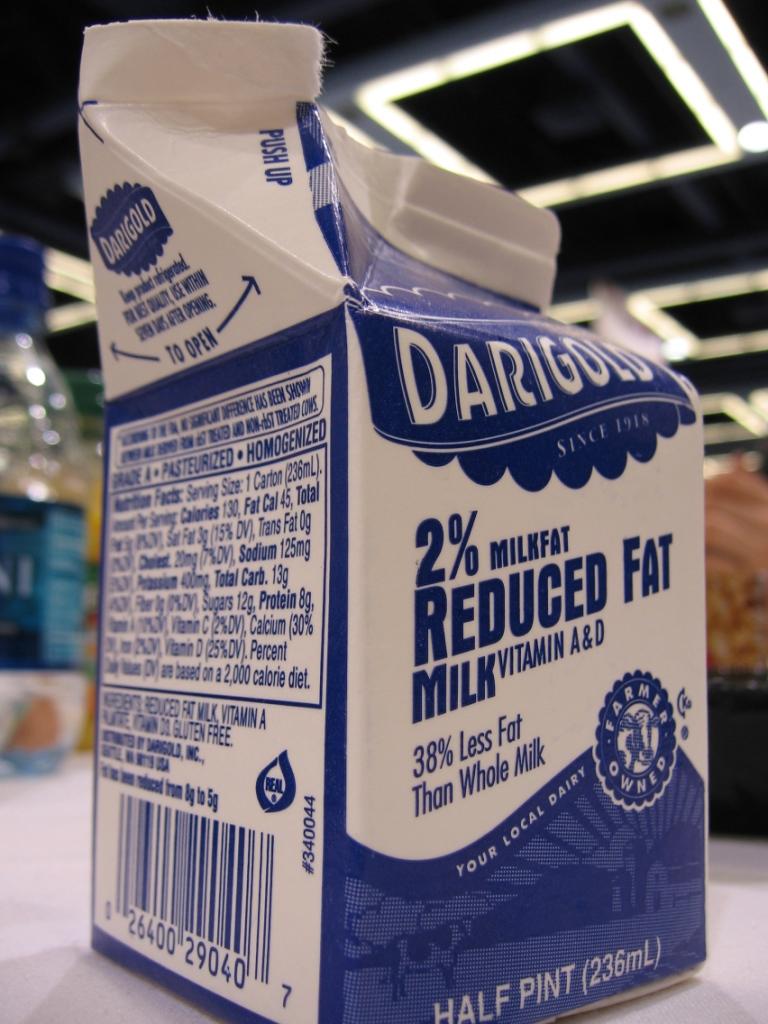The photograph captures a small, half-pint carton of milk prominently positioned on a white tabletop. The carton, adorned in blue and white, features the brand name "Dairy Gold" (D-A-R-I-G-O-L-D) set against a blue background in white letters. Below the brand name, the carton details its contents: "2% milk fat, reduced fat milk, vitamin A and D, 38% less fat than whole milk." It proudly declares "Since 1918" and "Your local dairy" in blue text, alongside a blue cow graphic, emphasizing its farmer-owned origins. The bottom of the carton reads "Half pint, 236 milliliters" in white against a blue background. The nutritional facts and ingredients are listed on the side, somewhat obscured due to the carton being tilted. The spout of the carton is open. In the background, a partially visible Dasani water bottle, slightly blurred, adds context. Above, you can discern a ceiling with some recessed square-shaped lighting fixtures, providing soft illumination in an otherwise dark space. The overall setting suggests the environment of a supermarket or similar establishment.